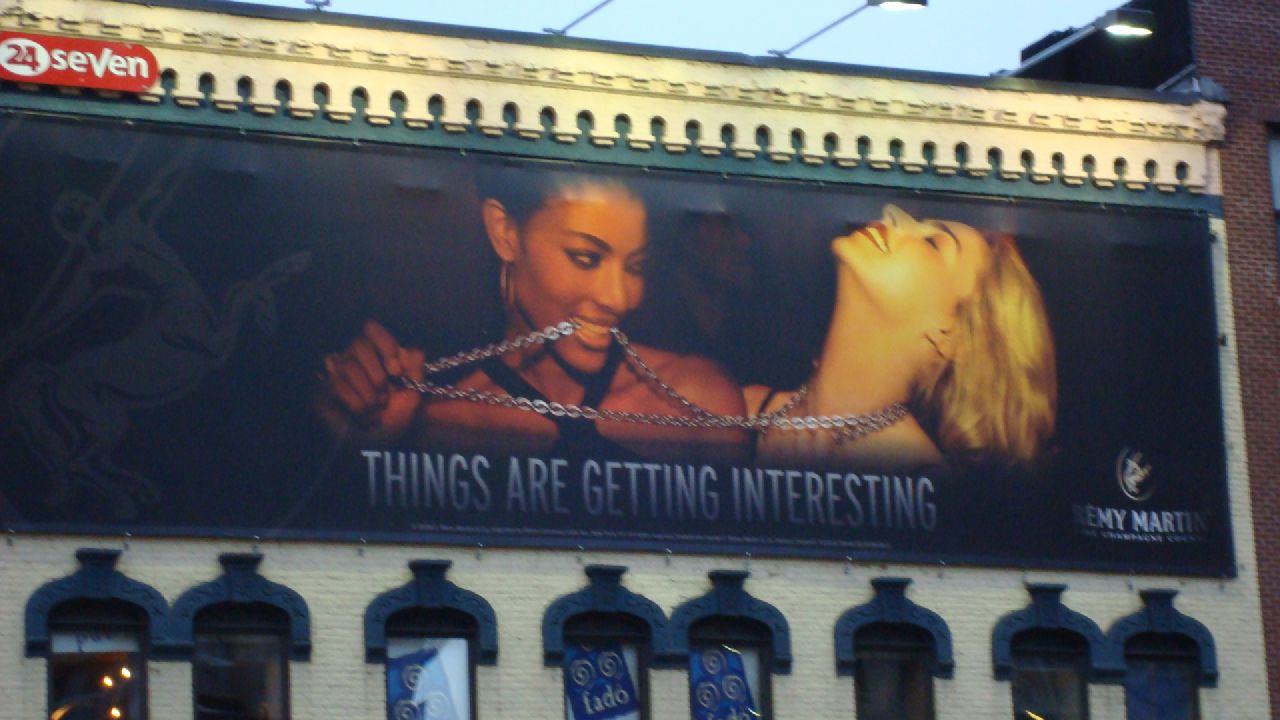The image depicts the exterior of a light beige brick building featuring a prominent billboard in the center. The building's façade includes eight windows, with the three central ones displaying a separate, striking blue advertisement that reads "FADO" in yellow swirls. The main billboard, lit by overhead lights, portrays two women in an intimate and joyful moment against a dark background. The blonde woman on the right has her head tilted back, laughing, while wearing a metallic chain necklace that the darker-skinned woman on the left playfully holds her mouth. The woman on the left also has her hair up in a bun and wears hoop earrings. The blonde woman dons red lipstick. The ad, seemingly for Remy Martin, includes the text "things are getting interesting" written in white ink. Additionally, a red "24-7" sign is visible at the top left corner of the image, enhancing the lively and dynamic scene.